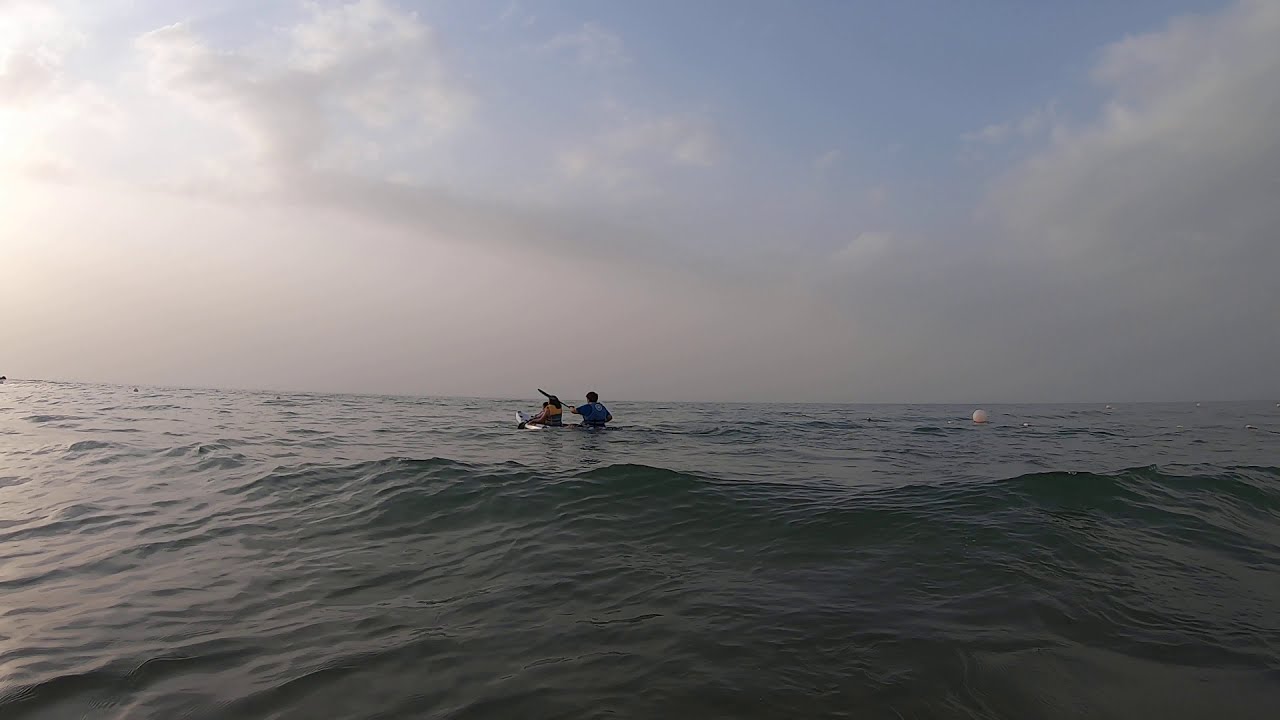In this captivating scene taken during the early evening, a white paddle boat with two people, a woman in the front and a man at the back holding the paddle, gracefully sails through a slightly wavy, grayish-blue ocean. Positioned in the center of the image, the pair appears to be steadily moving away from the forefront. The ocean, with its gray-green ripples, extends to the horizon where a faint, grayish-white foggy sky mixes with patches of blue. To the right of the boat, a white buoy ball floats gently on the water. The overall atmosphere is serene, with a backdrop of a vast body of water and a sky that hints at an impending sunset, casting soft light from the top left corner of the image.